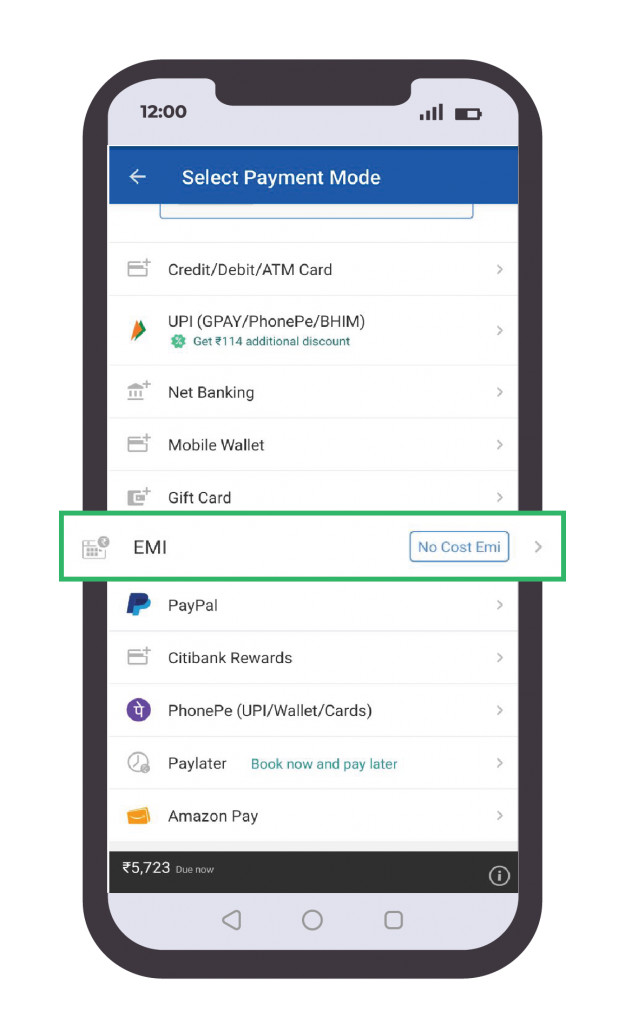The image depicts a mobile phone screen presenting a "Select Payment Mode" interface, showcasing a comprehensive list of payment options. The options include:

- Credit Card
- ATM/Debit Card
- UPI (like Google Pay and PhonePe BHIM)
- Net Banking
- Mobile Wallet
- Gift Card
- EMI and No-Cost EMI 
- PayPal 
- Citi Bank Rewards
- Pay Later
- Book Now & Pay Later
- Amazon Pay

The screen indicates an outstanding amount of 5,723 yen to be paid. The phone's status bar displays the time as 12:00, a battery at half charge, and full signal strength bars. This context suggests that the image is likely an instructional or promotional example, possibly demonstrating how to select an EMI option for payment. The organized list of payment methods and the specific UI details imply that it's designed to guide users through the process of selecting their preferred payment mode, emphasizing the No-Cost EMI option.